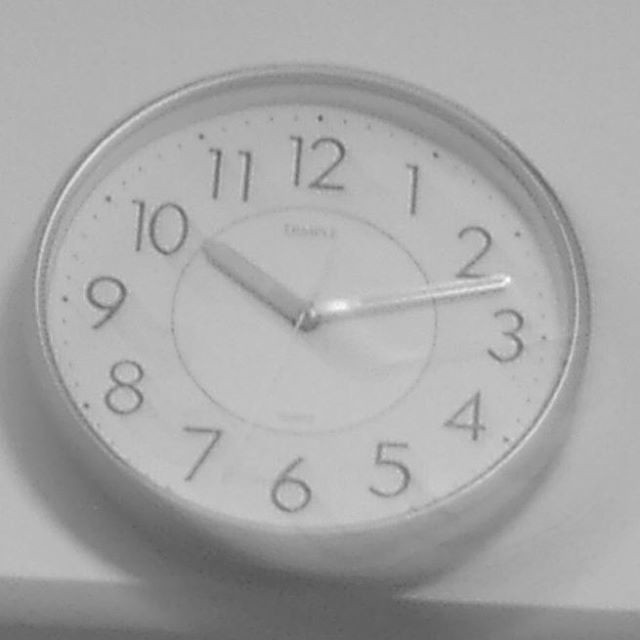The image features a detailed wall clock mounted against a white wall. The clock face includes the numbers 1 through 12, arranged in a clockwise sequence. Small dots mark the outer boundary of the clock face, adding a touch of elegance. The interior features a sophisticated, wound design encased in a sleek silver frame. 

The clock hands are positioned intricately; the minute hand points between 2 and 3, the hour hand rests at 10, and the second hand is caught between 6 and 7. At the center of the clock is a pristine white circular area, which contrasts with the brown inner circle surrounding it. The outer circle echoes the white theme, enhancing the clock’s polished appearance.

Silver reflections can be seen, likely owing to the clock's metallic elements, complementing the overall design. Shadows cast at the bottom give depth, suggesting overhead lighting. The entire clock face is protected by a clear glass cover, adding to its refined look.